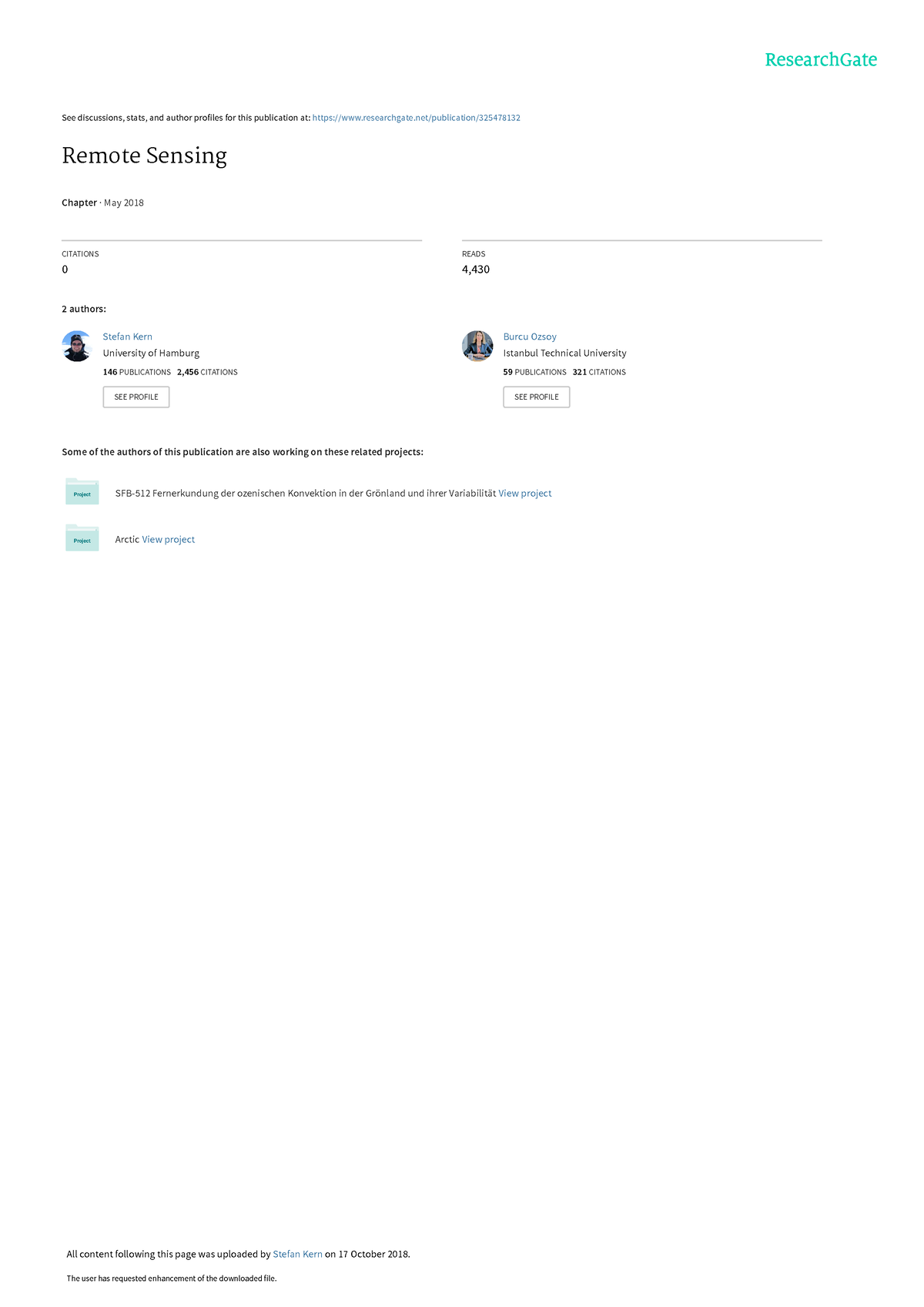In this highly detailed image, the top section features the heading, "See discussion stats and author profiles for this publication at ResearchGate.net/publications/325478132." The phrase "ResearchGate" is prominently displayed in turquoise on the right side. The largest text in the image is "Remote Sensing," situated below the heading. This is followed by the text "Chapter May 2018" accompanied by a gray horizontal line.

On the left, the section begins with "Citation 0," followed by details of two authors. The first author, "Stephen Kern," is highlighted in blue, with the affiliation "University of Hamburg" written below. Additional information lists "146 publications" and "2,456 citations," adjacent to which is a "See Profile" button.

To the right, the reads tally is "4,430." Below this, the second author, "Vercur Özsoy" from Istanbul Technical University, is listed with 59 publications and 321 citations, similarly accompanied by a "See Profile" button.

At the bottom, the image states that "Some of the authors of this publication are also working on these related projects:" followed by icons and titles of two projects. The first project, "SFB-512," is entirely in German. The second project, "Arctic-View," is displayed in blue.